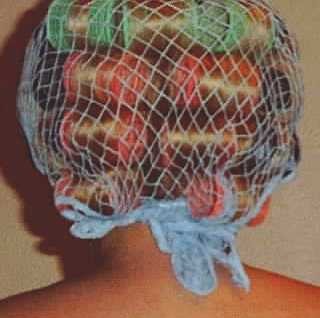The image captures a close-up, grainy digital photo reminiscent of a 1970s magazine. Dominating the frame from edge to edge, the shot focuses tightly on the back of a Caucasian woman's head and upper back, positioned against an off-gray, tan-hued wall. The woman's blonde hair is meticulously arranged in curlers: the top two are green, and the remaining six are red, spanning two vertical rows. Overlaying these curlers is a light blue, fishing-net-like bonnet with large diamond gaps. The ambient light creates a shadow on the left side of the wall, adding depth to the photograph.